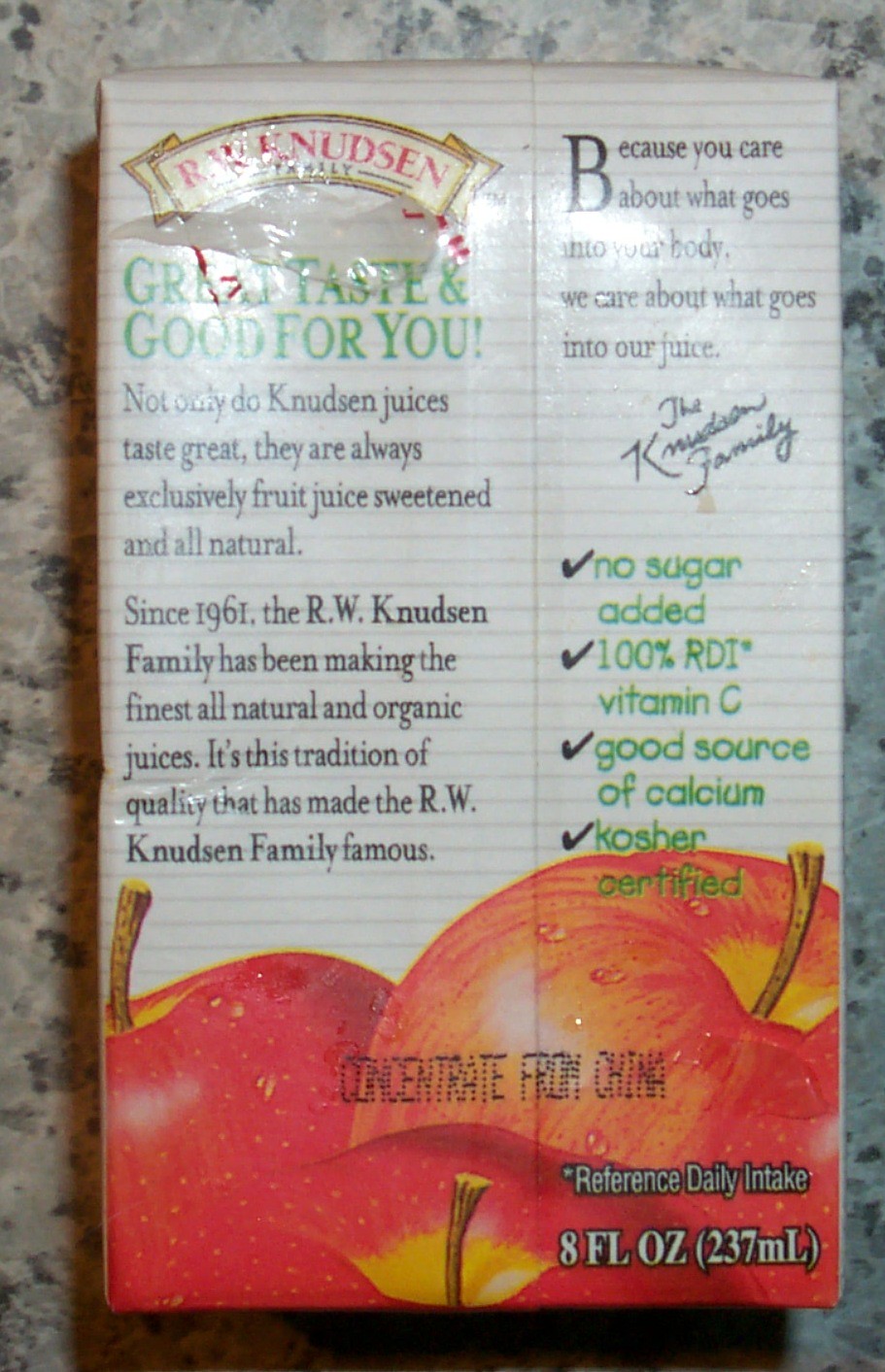This image features the back of a child's rectangular apple juice box, which is propped on a granite countertop exhibiting gray, white, light brown, tan, and black hues. The juice box itself has a predominantly white background adorned with light gray horizontal lines. At the top left, the brand name "RW Knudsen" is prominently displayed. A slogan in green, "Great taste and good for you," appears at the top right, followed by the phrase, "Because you care about what goes into your body, we care about what goes into our juice. - The Knudsen Family."

Below this, additional product claims are made, citing "no sugar added," "100% RDI of Vitamin C," "good source of calcium," and "kosher certified," all marked with checkmarks. At the bottom of the box, there are three large red apples, above which text indicates that the juice is from concentrate sourced from China. Further specific details include the volume specification of 8 fluid ounces (237 milliliters) located at the bottom right-hand corner along with a reference to daily intake of Vitamin C. This comprehensive array of information underscores the natural and health-focused qualities of the product, as well as the brand's longstanding tradition of producing all-natural and organic juices since 1961. There's some light reflection on the box, giving it a slightly wet appearance and adding a glare that makes it challenging to read the smallest print.